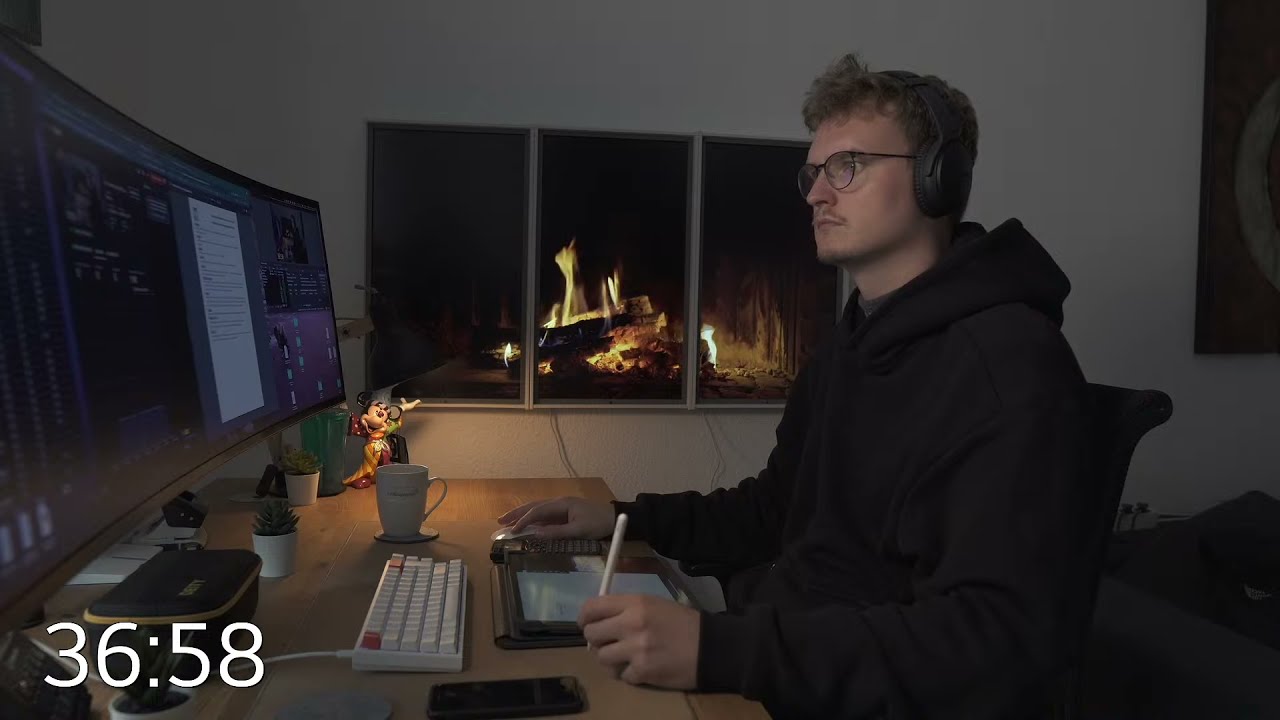In this image, a young man with short, dirty blonde, curly hair, wears eyeglasses, and black headphones. He appears to be deeply focused as he sits at a tan-colored wooden desk in a black office chair, staring intently at a large, curved computer monitor. Dressed in a dark hoodie, he holds a white stylus in his left hand, poised over a possible tablet. The desk is neatly organized, featuring a white keyboard, a coffee mug, a cell phone, and various small knickknacks. Behind him, on a white wall, hangs an animated picture mimicking a fireplace, adding a cozy yet modern touch to the dimly lit room. At the bottom left-hand corner of the image, the number 36.58 is visible. Although the screen content is not clear, the young man’s concentration suggests he might be working, browsing the internet, or getting ready to stream or play a game.